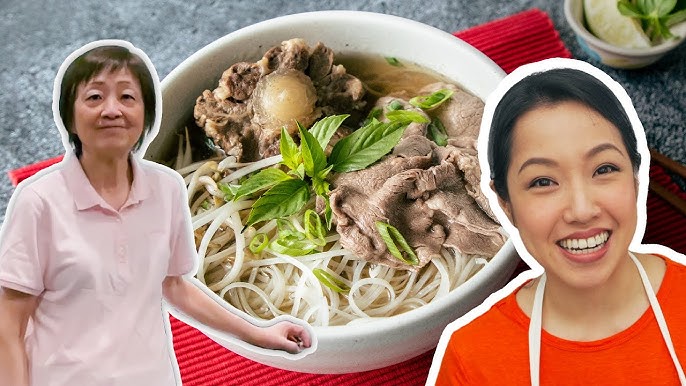This image is a detailed YouTube thumbnail or video thumbnail showcasing a Vietnamese pho recipe. Central to the composition is a vibrant bowl of pho, a traditional Vietnamese soup featuring a rich broth, noodles, slices of meat, and garnished with chopped green onion and other vegetables. The soup is presented in a white bowl placed on a red placemat on a gray and light gray speckled table, beside a cup.

Superimposed on this culinary centerpiece are two separate photographs of Asian women. On the left is an older woman with ear-length dark hair, wearing a light pink shirt. She has a moderate smile and her hand appears near the bowl of soup, though it's clear she is not in the same physical space as the dish. On the right is a younger woman with red lipstick, perfectly groomed eyebrows, and her hair pulled back. She smiles broadly, showing both her top and bottom teeth. She's dressed in an orange-red shirt and appears to be wearing a kitchen apron, suggesting a culinary role.

The overall image effectively blends the appetizing allure of the pho with the warm, engaging presence of the two women, hinting at a personal connection or family tradition behind the recipe.